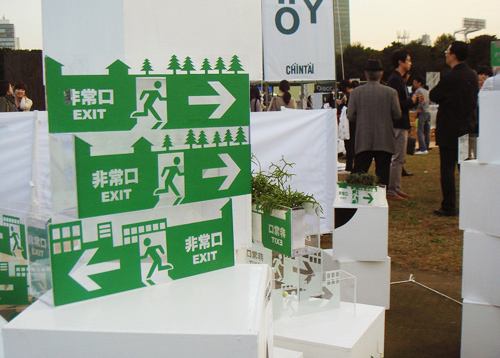The image depicts an outdoor event held in a grassy park setting. In the foreground, there is a prominent white, glossy, square-shaped platform that narrows towards the top, displaying a plastic sign on top. This sign features three distinct, vertically stacked green signs, each illustrating a running stick figure exiting through a doorway. The top two signs have arrows pointing to the right, and the bottom sign has an arrow pointing to the left, all accompanied by the word "Exit" in English and Chinese characters. The background reveals multiple kiosks and booths, as well as people mingling among them, with the sky and trees visible in the distance. The individuals are mostly facing away from the camera, suggesting they are engaged in conversation or observing the displays. The overall scene takes place in the daytime, capturing the lively atmosphere of the event.